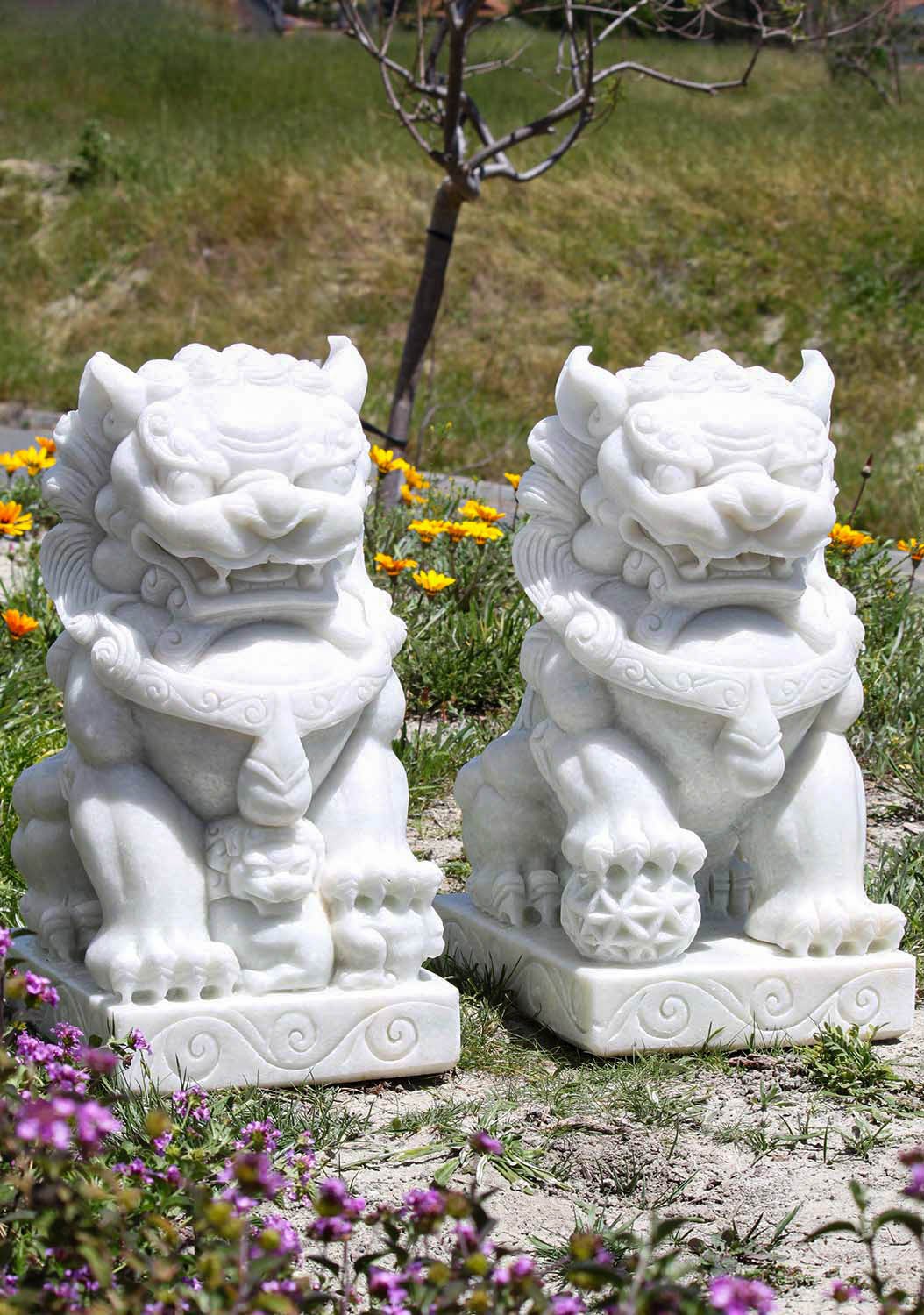The image showcases an outdoor garden scene dominated by two large, intricately detailed Asian-style lion statues made of a white marble-like material. The statue on the left features a lion with its left paw resting on a ball, and a smaller lion figure situated between its front legs. The statue on the right mirrors this design, with its right paw atop a sphere. Both statues bear open-mouthed expressions, displaying their teeth, and are adorned with chains or necklaces embellished with hanging jewels. They stand on plinths, resembling bookends that frame the scene. The garden setting is vibrant with a foreground of purple flowers and background bursts of yellow and orange blossoms, complemented by a stretch of green grass and patches of exposed sandy-gray soil. The overall composition is bathed in bright sunlight, creating a lively and colorful atmosphere.